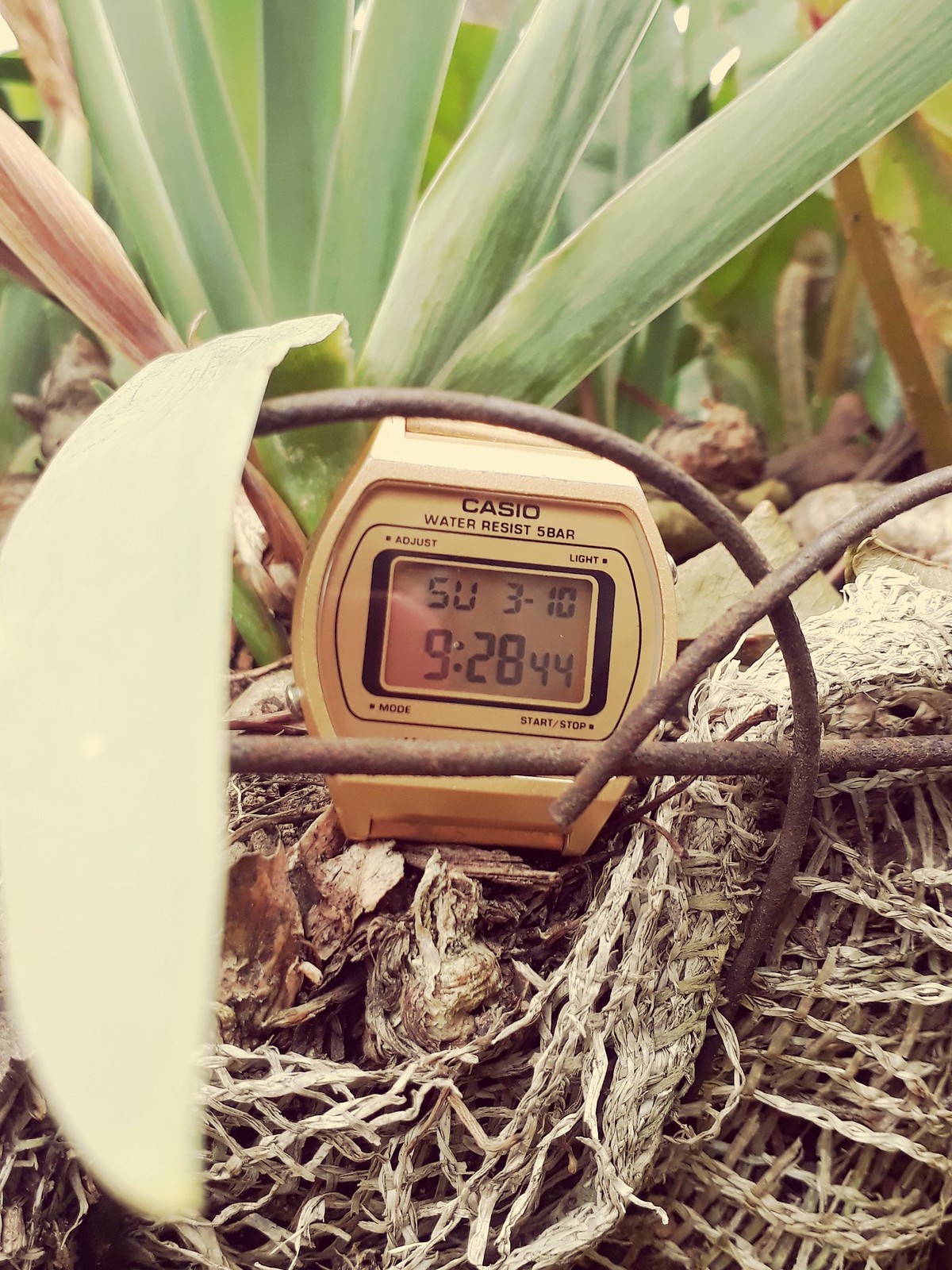The image showcases a Casio wristwatch prominently displayed outdoors against a backdrop of partially visible green plants with long, straight, flat leaves resembling those of a succulent. The watch is set within a round metal frame extending into a long section on the right. The metallic frame houses the gold-colored Casio watch, which features a gold rectangular face bordered in black, with black numbers. The watch face is also marked with the code "92844SU3-10." Below the watch is a light tan or brown material that appears to be burlap or netting. Adding a touch of contrast, a yellow-tinged leaf from the plant bends down over the metal piece on the right-hand side.